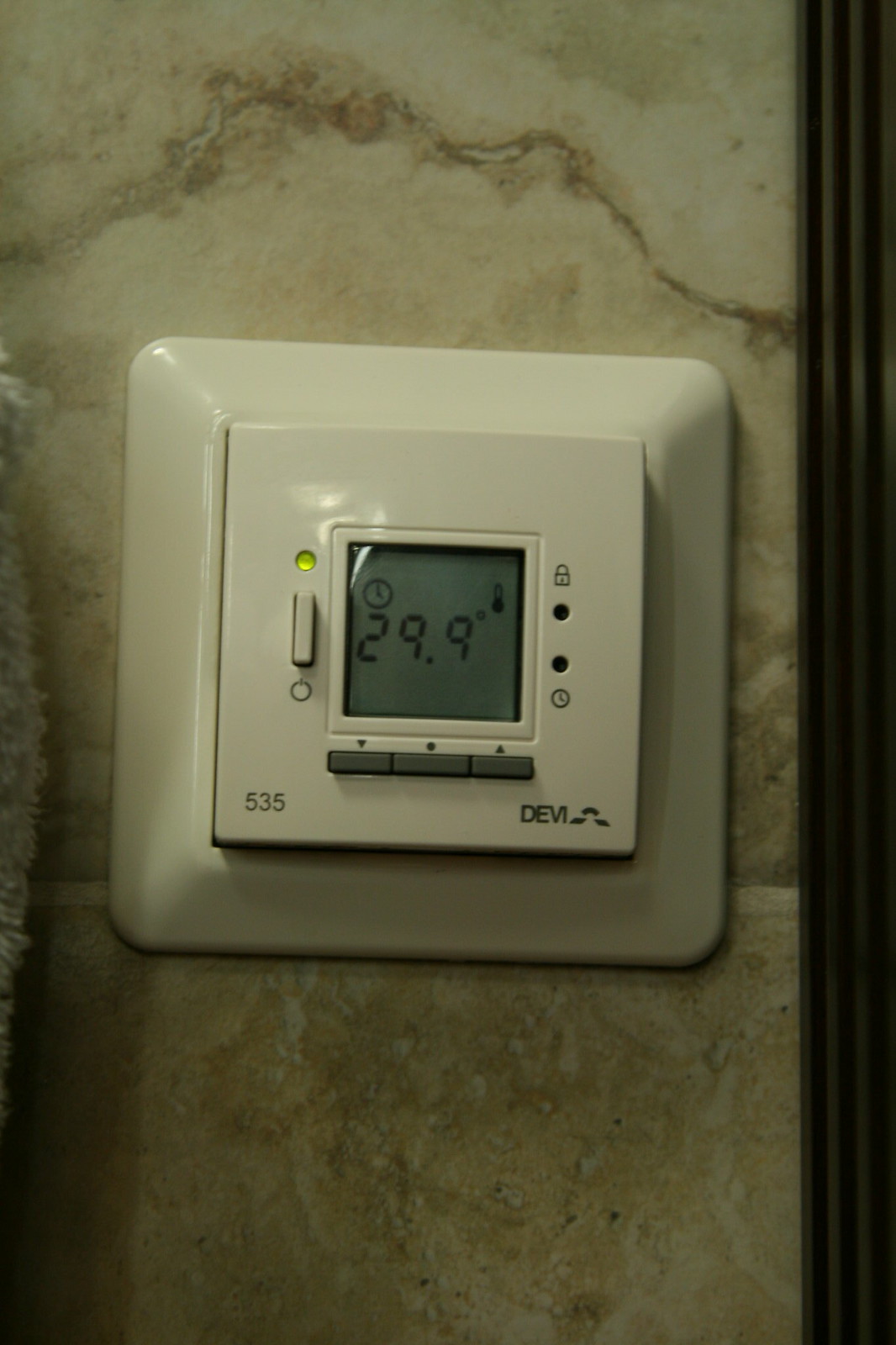A close-up image depicts an old-fashioned thermostat mounted on a marble wall, possibly in an apartment building. The thermostat, made of beige-white plastic, appears slightly tilted to the right but is otherwise centered in the frame. Despite the dim lighting and somewhat blurry quality of the photo, several details are discernible. The digital display on the thermostat reads 29.9 degrees Celsius, with a clock icon situated just above the temperature reading and a temperature icon further to the right. The device is branded "DEVI," identifiable by a logo resembling a small pyramid, and is marked with the model number "535" at the bottom. Although several indicator icons exist above unlit lights, a green light is illuminated, signifying that the thermostat is currently operational.